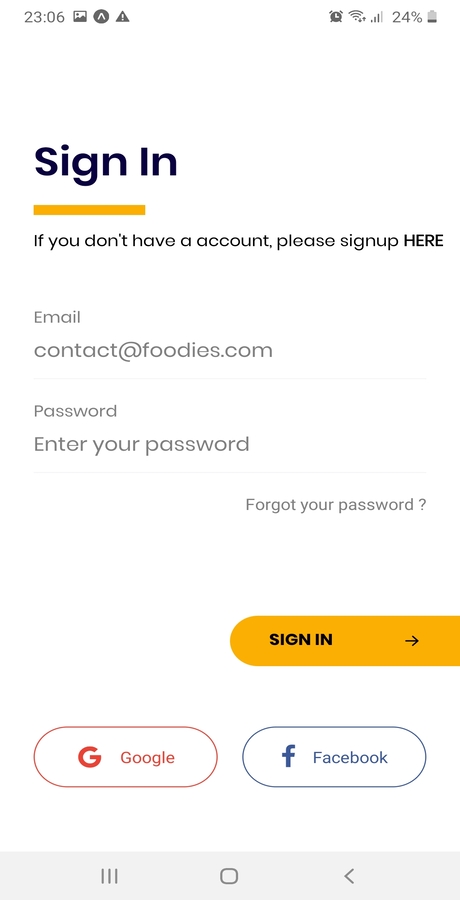The image is a screenshot of a sign-in page for a website. On the left side, positioned towards the middle, there is a bold heading that reads, "Sign-In." Directly below this heading, there's a prompt stating, "If you don't have an account, please sign up here." Beneath that is a field label that says "Email," instructing users to contact "contact@foodies.com" for assistance. Following this, there's a "Password" field labelled "Enter your password." On the right side of the password field, there is a clickable text that reads "Forgot your password." 

Underneath these instructions, a prominent yellow button is displayed with the text "Sign-In." Additionally, there are two alternative sign-in options: a button on the left side labeled "Google" and another button on the right side labeled "Facebook." At the bottom of the page, there are three navigation buttons: a "Home" button, a "Back" button, and a "More" button, providing further navigation options for the user.